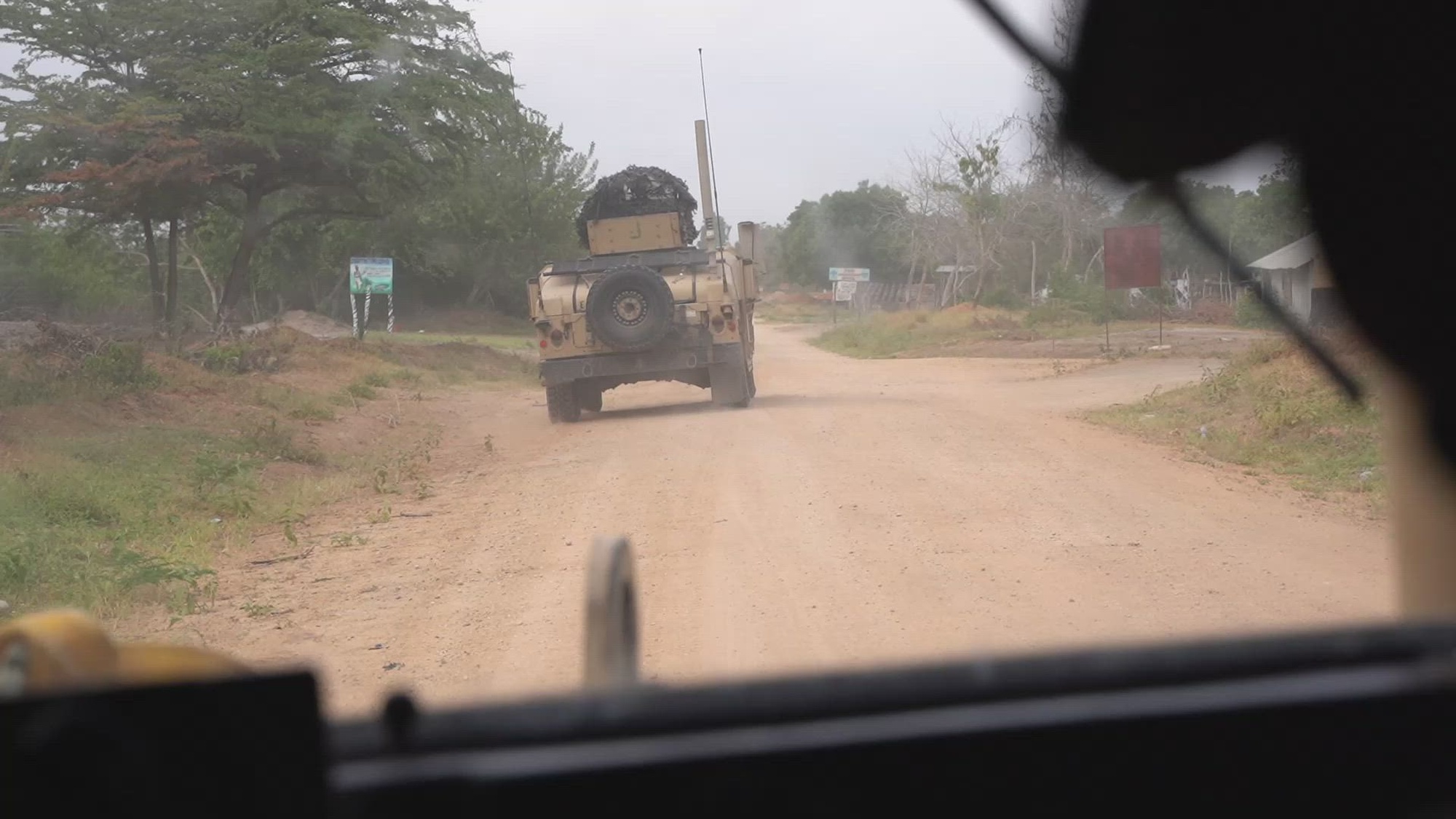The photo captures the view from within a vehicle, looking out through the windshield onto a sandy, dirt road. The vehicle ahead appears to be a tan-colored military SUV, possibly a Humvee or a similar type, equipped with a tall antenna, a large spare tire mounted on the back, and what seems to be a covered gun turret or a viewing cage on top. This vehicle is traveling along a route flanked by sparse trees and minimal grass, giving the impression of an abandoned or war-torn area. In the distance, green foliage is evident along the road's shoulder. Numerous unidentifiable signs dot the surroundings, including a red sign towards the right and a multicolored sign on the left. The sky is overcast, casting a dull, grey hue over the scene, further accentuating the desolate ambiance. The photograph is distinctly taken from behind the windshield of another heavy-duty vehicle, potentially implying involvement in some form of military convoy or excursion.